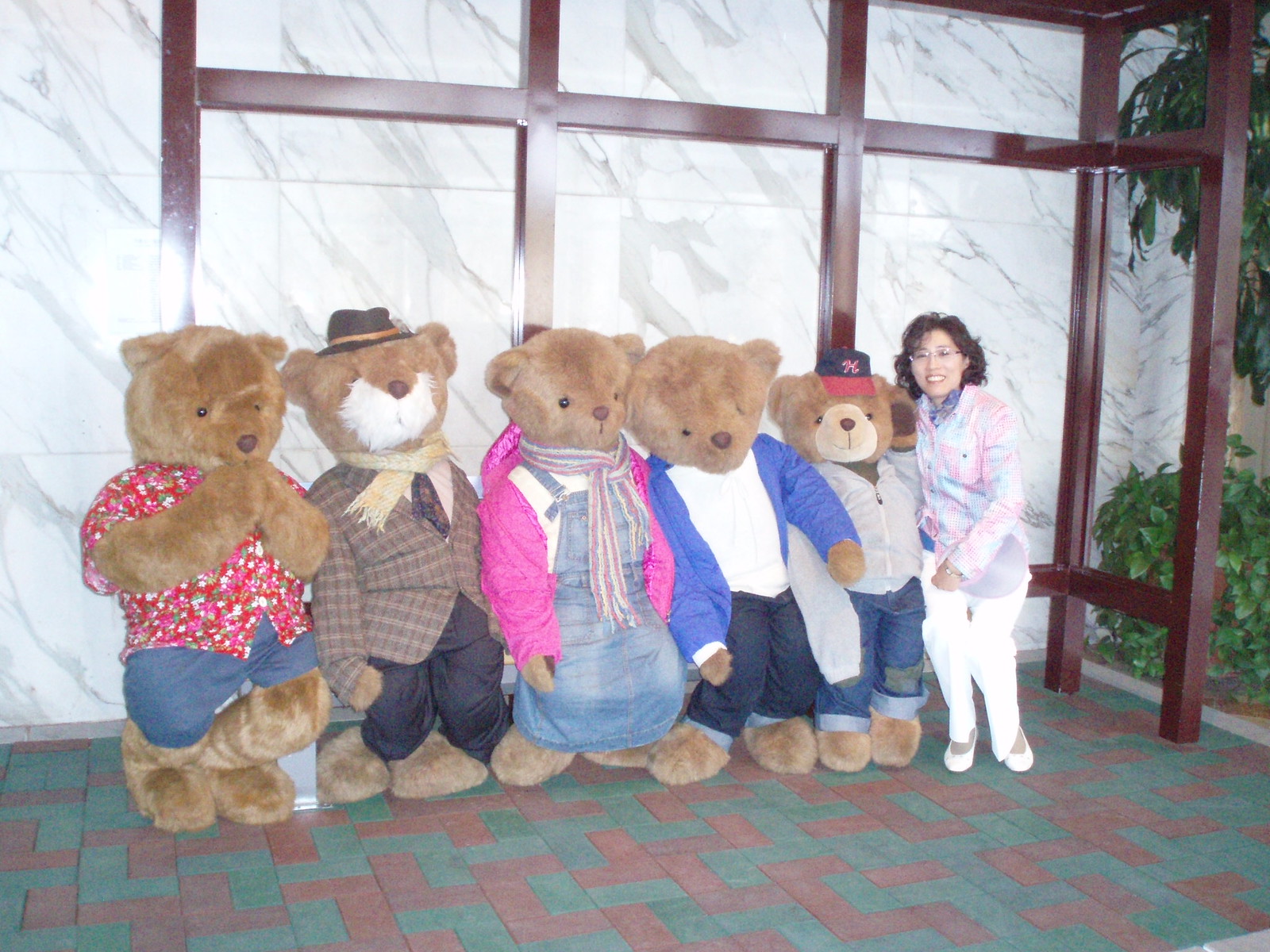This photograph captures an Asian woman with black hair and glasses, smiling as she poses with five human-sized teddy bears. The scene is set outdoors in front of a striking white marble wall veined with gray. Multicolored brick tiles—red and green—pave the area beneath the bears, which appear to be leaning against a wooden beam structure. In the background, one can spot a lush green bush and the leaves of a tree.

Each life-size bear is uniquely dressed, adding character to the whimsical scene. From left to right:
1. The first bear sports a red and white floral shirt paired with blue shorts.
2. The second bear, looking distinguished, wears a brown checkered coat, a black tie over a white shirt, black pants, a brown scarf, and a dashing hat. Its face features a white beard-like pattern, giving it an older appearance.
3. The third bear, dressed in feminine attire, has on a pink jacket over a white shirt, a blue denim jumper, and a pink and white striped scarf.
4. The fourth bear wears a blue jacket, a white shirt underneath, and blue jeans.
5. The fifth bear, adorned with a red and black baseball cap, a grayish sweater, and cuffed blue jeans, stands beside the woman.

This delightful assembly of clothed teddy bears and the woman's joyful presence creates a charming, picturesque moment.